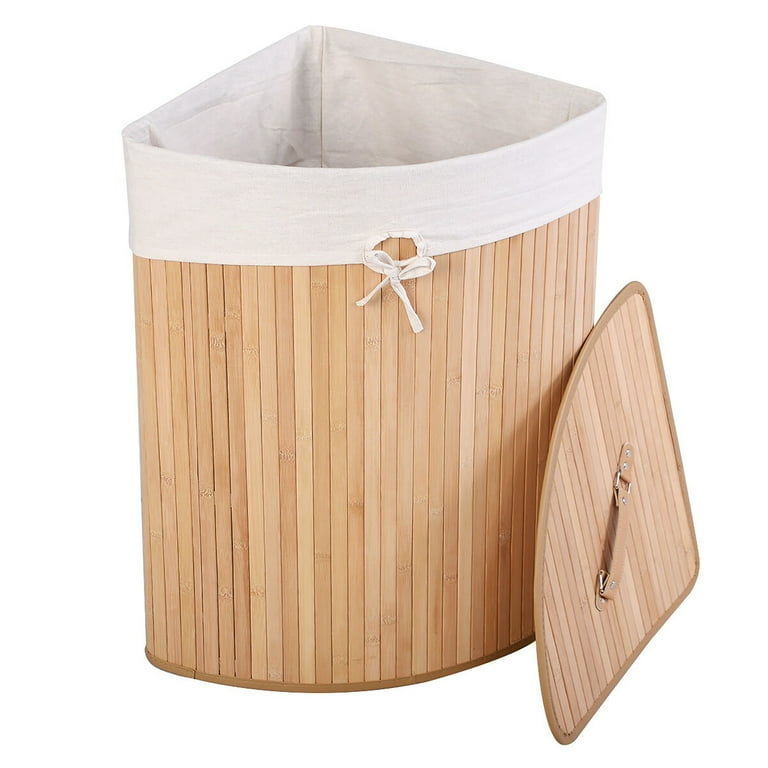This is a detailed product image of a triangular-shaped clothes hamper designed to fit snugly into a corner. Crafted from light brown wood, the hamper features vertically connected thin wooden slats. The front of the hamper is curved while the back comes to a sharp point. The lid, which matches the hamper’s triangular shape, is currently positioned leaning against one of the front corners. Both the lid and the hamper are equipped with brown leather handles for ease of use. Inside the hamper, there is a removable, washable white fabric liner that is secured with a string tie at the front. The entire setup is displayed against a completely white background, emphasizing its clean and elegant design suitable for any closet or corner space.